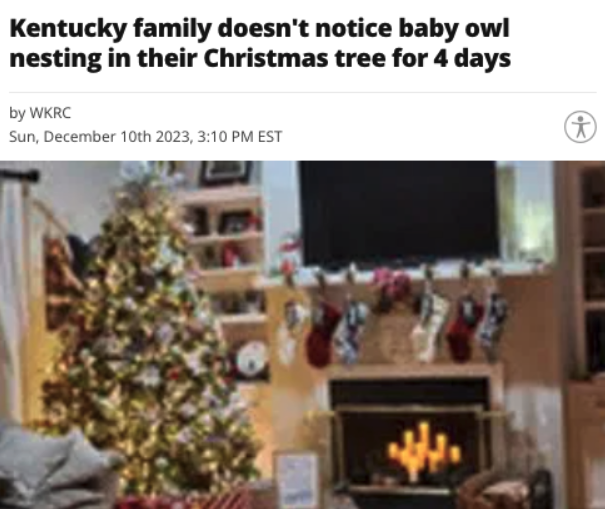This image captures a news story headline: "Kentucky Family Doesn't Notice Baby Owl Nesting in Their Christmas Tree for Four Days," prominently displayed in bold black text at the top. The story is attributed to WKRC, with smaller black text indicating the date and time as Sunday, December 10th, 2023, at 3:10 p.m. Eastern. To the right, there is an emblem of a stick figure enclosed in a circle against a white background.

The lower portion of the image is dominated by a blurry photograph depicting a cozy living room. On the left side, a Christmas tree stands, partially obscured, with a bookcase behind it filled with various items. A television is mounted above a fireplace mantle, which is decorated with stockings. Inside the fireplace, candles are lit, adding a warm glow to the scene. The right side of the image suggests the presence of another bookcase, creating a symmetrical setting with the TV and fireplace centered between the two bookcases. Although the clarity is lacking, the photo hints at a bright daylight setting. Notably, the baby owl mentioned in the headline is not visible in the image.